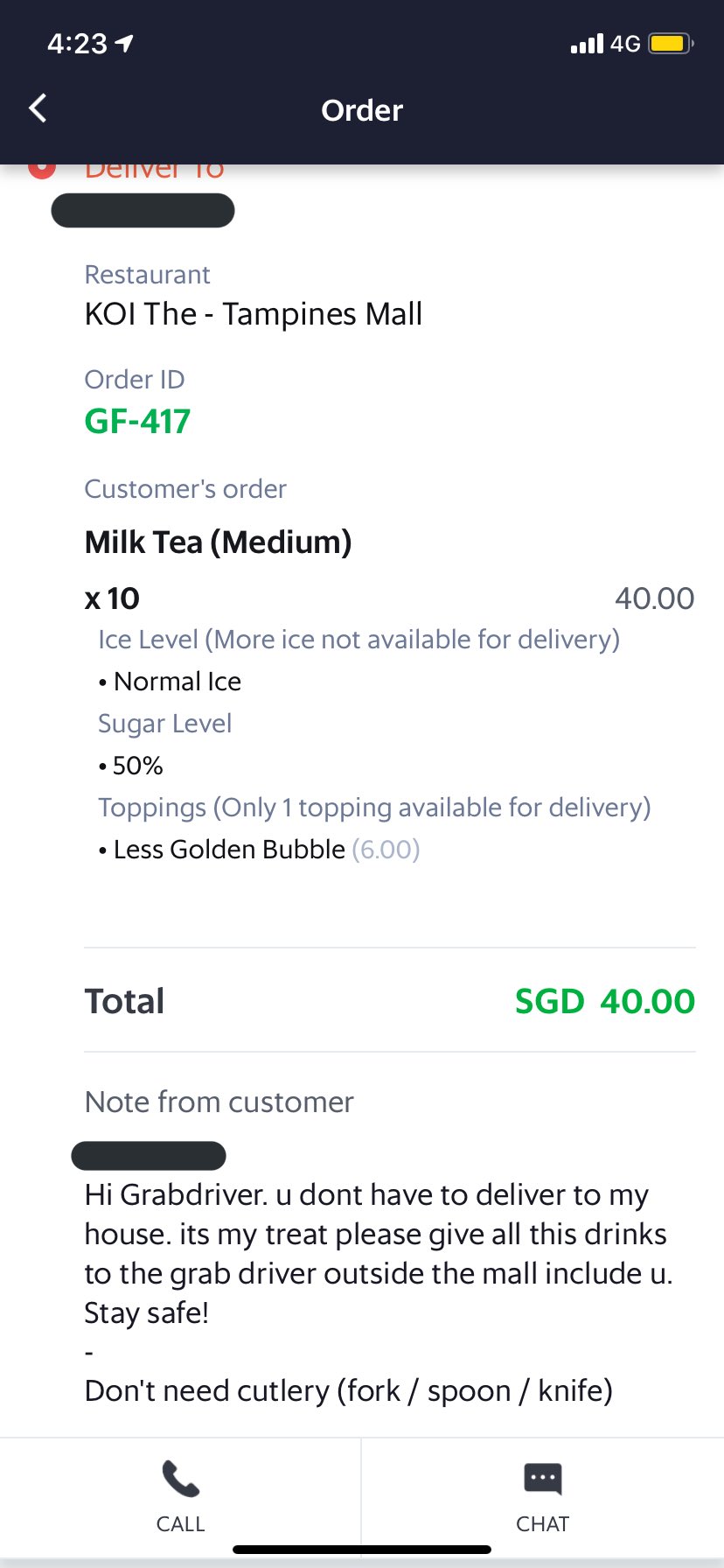**Screenshot Description:**

The screenshot features an order summary from a restaurant named KOI located in Tampines Mall, displayed on a white background. The Order ID is highlighted in green as GF417, and it belongs to a customer who ordered 10 medium-sized milk teas, priced at $40 in total. The milk teas have specific customizations: the ice level is set to "more ice," and since "more ice" is unavailable for delivery, "normal ice" is indicated in bold. The sugar level is specified at 50%, also in bold. For toppings, only "less golden bubble" is available for delivery, presented in bold text as well. The order's total cost is SGD $40, marked in green.

A note from the customer, partially blacked out, addresses the Grab driver, stating, "Hi Grab driver, you don't have to deliver to my house, it's my treat. Please give all these drinks to the Grab driver outside the mall. Stay safe!" This message emphasizes the customer’s kind gesture. Additionally, there's a note indicating that cutlery (fork, spoon, knife) is not needed.